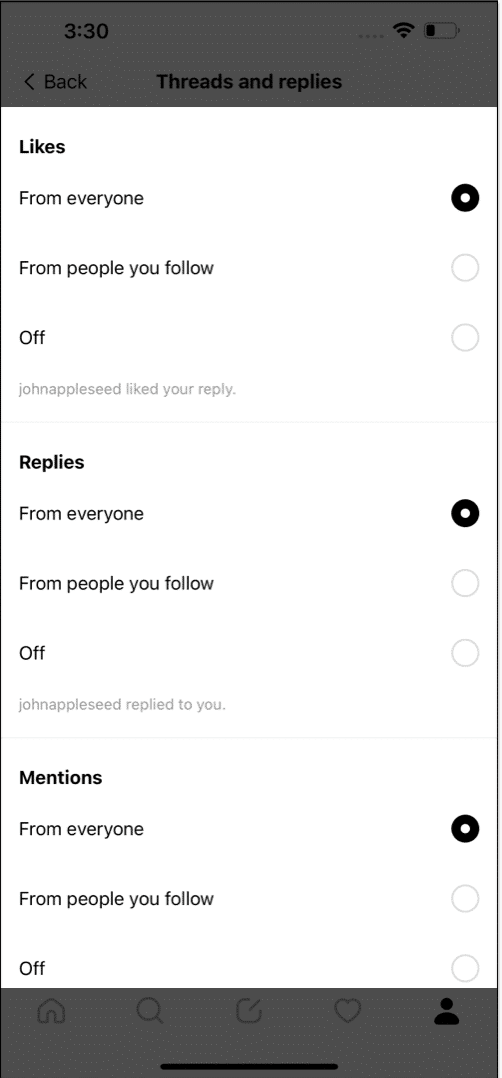The image showcases a smartphone screen with the battery at 25% and a strong Wi-Fi connection. The time displayed on the device is 3:30. The top section of the screen is titled "Threads and Replies," highlighted in a gray background. Below this, three categories are presented: "Likes," "Replies," and "Mentions."

In the "Likes" category:
- Notifications for "From Everyone" are turned on.
- Notifications for "From People You Follow" and "Off" are both turned off.
- A message reads, “John Appleseed liked your reply.”

In the "Replies" category:
- Notifications for "From Everyone" are active.
- Notifications for "From People You Follow" and "Off" are both inactive.
- A message states, “John Appleseed replied to you.”

In the "Mentions" category:
- Notifications for "From Everyone" are enabled.
- Notifications for "From People You Know" are turned off.
- The "Off" option is also off.

At the bottom of the screen, a shaded navigation bar features icons for a person, a search bar, a clock, a home, and a message, offering various functionalities for the user.